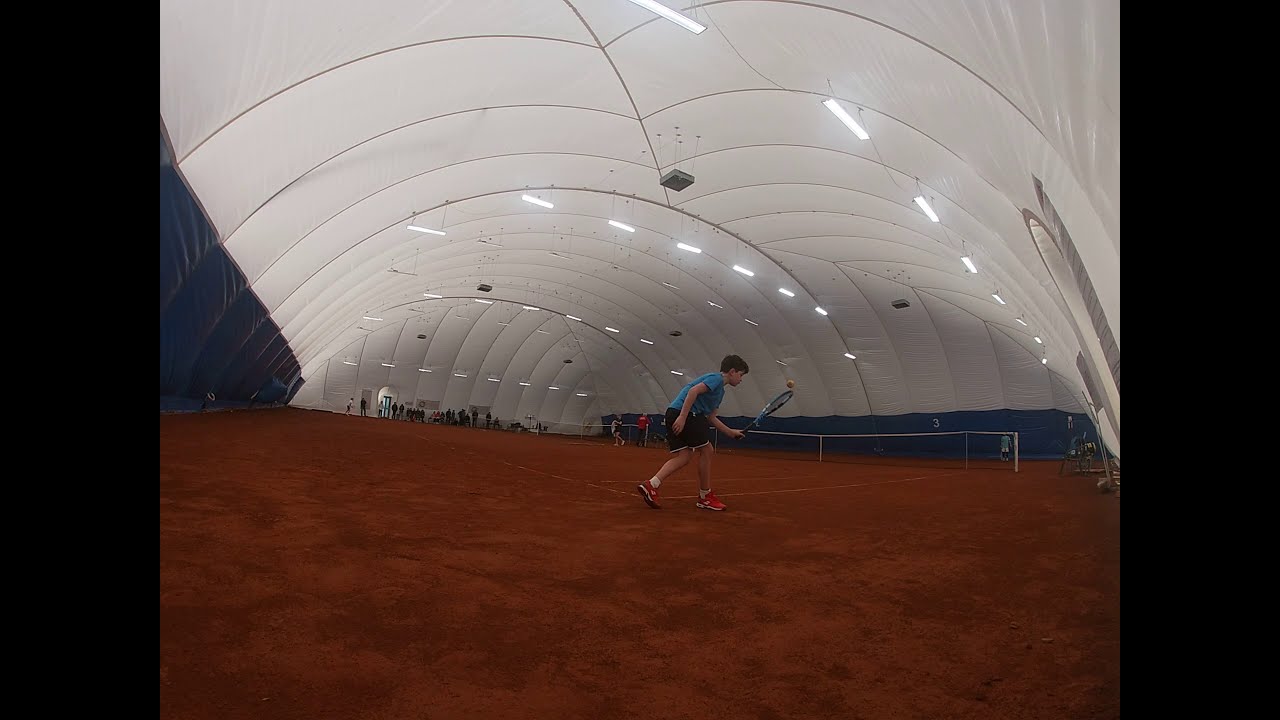In the image, we see an indoor tennis facility that resembles a large, tent-like structure with white, scalloped ceilings illuminated by overhead lights. The ground is covered with dirt. At the forefront, a young man, likely a teenager, is playing tennis. He is poised to hit the ball, wearing a light blue t-shirt, dark blue shorts, and red tennis shoes. In front of him stands a tennis net. To the left of this net, another tennis court is visible, where a couple of other players are playing. Beyond this second court, there is a line of people sitting. The tent structure features additional hanging equipment, possibly air conditioners. The edges of the tent near the ground have blue borders.